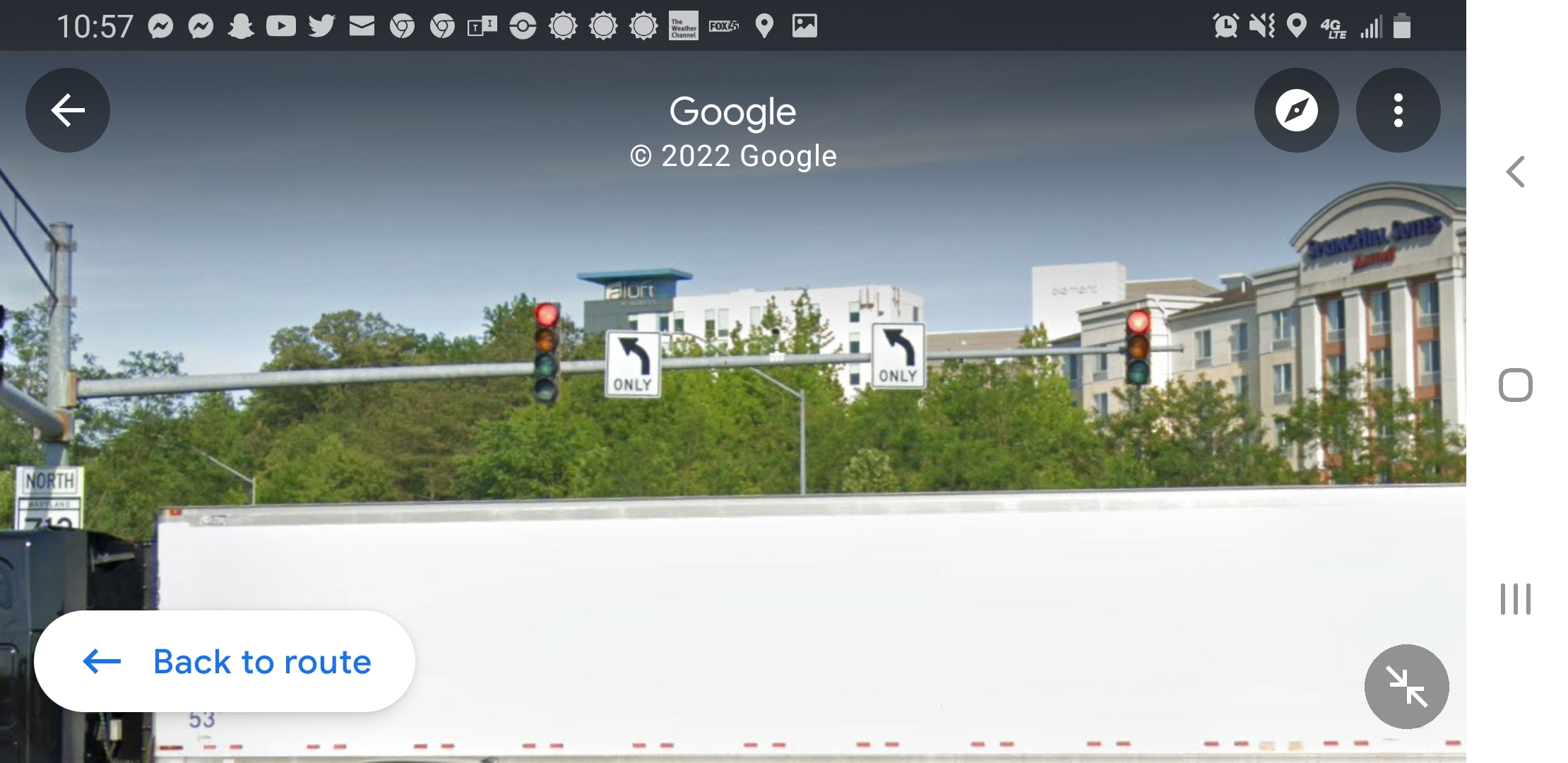The image is a color photograph capturing the screen of a laptop displaying Google Earth. At the top of the screen, there is a black bar indicating the time as "10:57," along with a series of various icons. Some of these icons include familiar ones such as Snapchat, Twitter, email (envelope), Google Chrome (multicolored circle), and others like a camera shutter symbol, cogs, and an alarm clock icon. More icons, including a speaker icon that is crossed out (indicating the sound is off), a pin locator similar to Google Maps, a 4G signal indicator, a signal strength icon, and a battery icon, are also visible.

The photograph depicts a clear, detailed aerial view of an intersection, possibly from Google Earth. Several elements are prominent: a large building that looks like a bank on the right, multiple buildings, traffic lights, two left-turn lanes with vehicles waiting at red lights, and a row of trees lining the streets. Additional features include a highway sign on the left indicating a direction "North" and an oblong blue button on the bottom left of the screen labeled "Back to Route," suggesting there's a way to return to the guided path. In the bottom right corner, there's a circle with arrows pointing towards each other, likely a control for zoom or navigation within the map interface. The footer of the screen verifies the source with the text "Google" and "© 2022 Google".